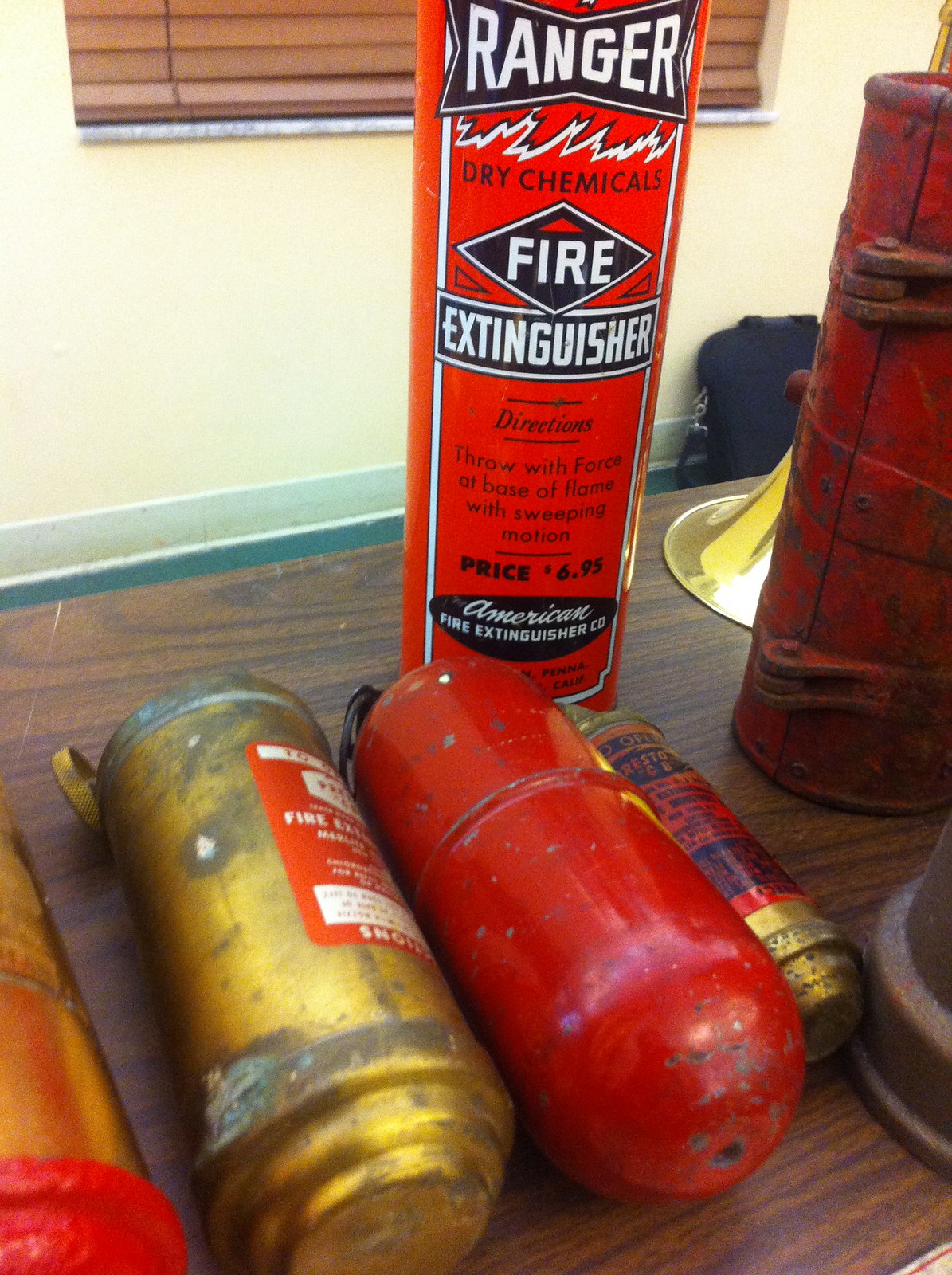The image, taken indoors, shows a wooden table in what appears to be a standard room with pale yellow or cream-colored walls and old brown blinds drawn over a window. Leaning against the wall on the floor is a black laptop bag. On the table, which resembles an older desk, there are several canisters that look like fire extinguishers. Prominently, a bright red extinguisher stands upright, bearing the label "Ranger Dry Chemicals Fire Extinguisher," with directions stating, "throw with force at the base of flame with sweeping motion," and priced at $6.95. The label further identifies it as a product of the American Fire Extinguisher Company. Alongside this extinguisher, lying down on the wooden surface, are additional old-style metal cylinders—one gold with a red label and another red with a black handle, both appearing slightly worn. The scene is framed by a mundane backdrop, enhancing the focal display of these vintage fire safety devices.